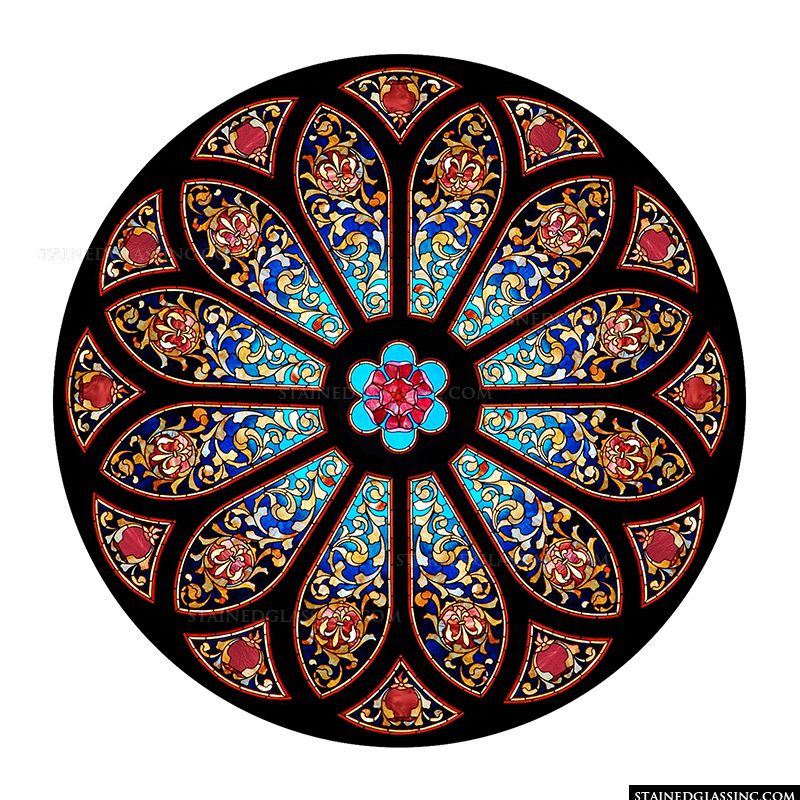This is a detailed photograph of an intricately designed circular stained glass window, possibly from a church or a ceiling dome, created by stainedglassink.com. The design is centered around a flower motif, with petals crafted from blue stained glass interspersed with intricate patterns. Each petal features a cascading semicircle design resembling seashells, transitioning from blue to beige in repeating patterns. Within each petal, suns or sun-like symbols represented in orange and beige colors are spaced out with black lead lines. At the very center of the flower is a black lead circle encasing a smaller flower-like design. This inner flower has cyan petals with red secondary petals and a red core. Surrounding the flower, fanned-out triangles with pear-shaped brown objects are positioned upside-down to complete the composition. The overall piece incorporates colors such as blue, red, gold, yellow, orange, and black, and is marked with the gray text "stainedglassink.com" at the bottom right corner, suggesting the photograph was taken to showcase their craftsmanship.